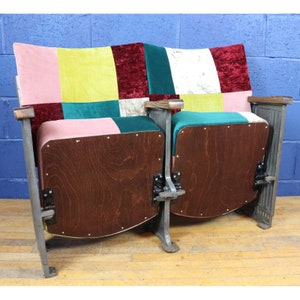The image showcases a pair of modified, side-by-side theater seats sitting on a pine-like, wooden gymnasium floor. The floor is unvarnished and resembles something you might find in an old-style gym. Behind the seats, there is a wall composed of large, blue-painted bricks, imparting a noticeable contrast to the more vibrant chairs. 

The theater seats are spring-loaded, with the cushions folded upright, requiring manual adjustment to sit. Each chair has an armrest, with a shared one in the middle, signifying their original theater use. The upholstery is a rich, velvety fabric adorned with a patchwork of colorful squares. These squares are roughly seven inches each and feature a whimsical array of colors including pink, red, yellow, burgundy, turquoise, lime green, and white, giving the chairs a retro 70s or 80s vibe. Despite their vintage appearance, the chairs are in excellent condition. They are not fastened to the wooden floor, allowing for easy placement and arrangement. The overall scene strikes a balance between the old and new, with a unique artistic flair.